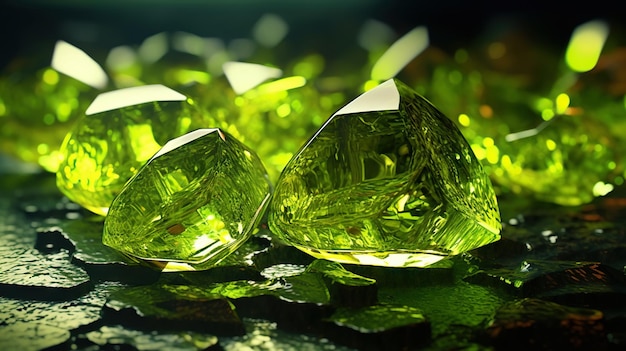The image is a close-up shot of vividly green gemstones, likely emeralds, arranged on an uneven, glossy surface that has light glistening off it. The two most prominent gems are centrally positioned, exhibiting a crystalline, hexagonal form with a brilliant gleam. Surrounding these are additional gemstones, slightly blurred towards the left and receding into the background. These gem structures appear layered and arranged in rows, showcasing a range of clarity and blurriness as they extend backwards. The surface they rest on is similarly green and has a somewhat gelatinous appearance, enhancing the overall vibrant emerald hue. Light shines from the top-left, casting reflections and a soft glow across the stones, making the scene sparkle. The gemstones possess clear cubic cuts and display their internal veins and structure, giving the viewer a detailed look into their crystalline beauty.